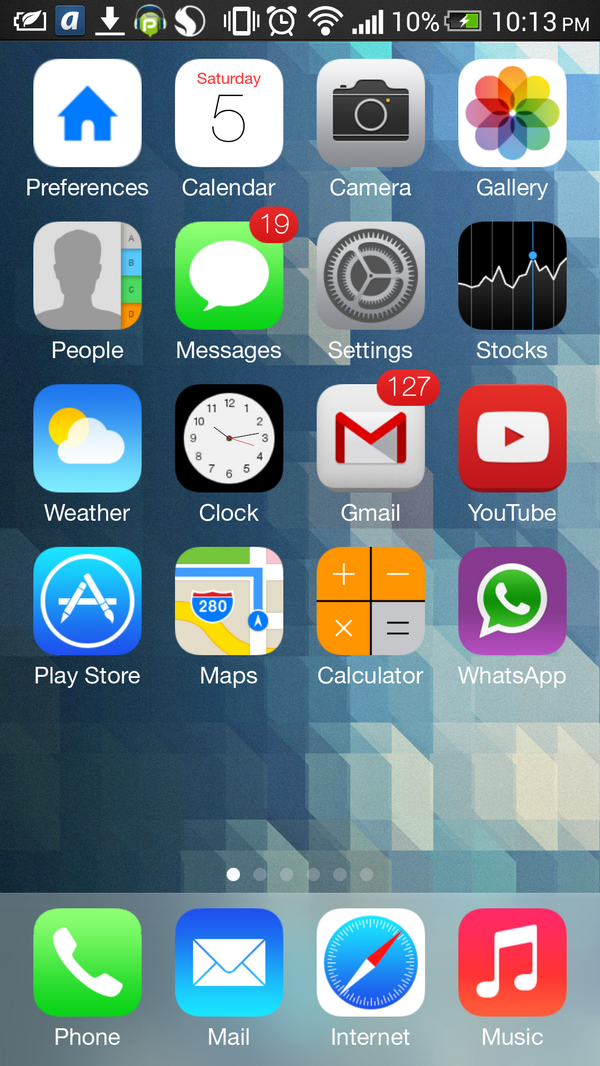**Detailed Caption:**
The screenshot captures the homepage of a mobile phone with a sleek and modern aesthetic. The background features a geometric design predominantly in shades of white, gray, and blue. At the top, there is a black status bar containing various icons lined up in a single row. The top right corner displays the time "10:13 PM" in white text. 

Below the status bar, the main section of the screen displays rows of app icons, each accompanied by a label in white text. The first row includes (from left to right): 
1. Preferences
2. Calendar
3. Camera
4. Gallery 

The second row features: 
1. People
2. Messages
3. Settings
4. Stocks

The third row includes: 
1. Weather
2. Clock
3. Gmail
4. YouTube

The fourth row showcases: 
1. Play Store
2. Maps
3. Calculator
4. WhatsApp

At the bottom of the homepage, there are six navigation dots indicating the number of home screens; the first dot is white, signifying the current screen, while the remaining five dots are gray.

Just beneath the navigation dots, there is a semi-transparent pane that slightly blurs the background design behind it. This pane contains four primary icons, each with its respective label in white text:
1. A green square with a white phone icon labeled "Phone."
2. A blue gradient square with a white envelope icon labeled "Mail."
3. A white square with rounded corners featuring a blue compass icon, labeled "Internet."
4. An orange to red gradient square with white musical notes icon labeled "Music."

The overall layout is clean and organized, with a distinct modern touch to the visual elements.